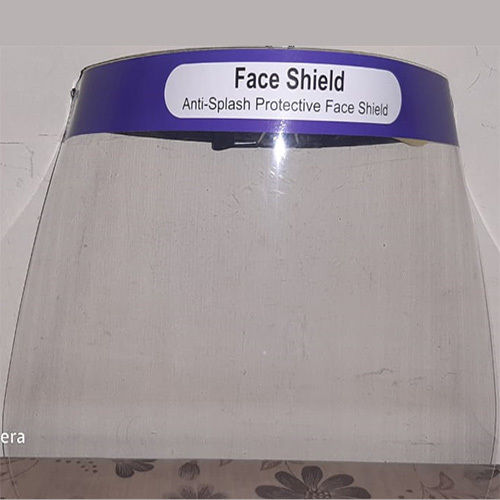The image showcases a large, clear plastic face shield prominently displayed against a very light gray background. The face shield features a blue or purple top band, which is adorned with a white label. The label, written in black text, reads "Face Shield" in bold lettering, followed by "Anti-Splash Protective Face Shield" in regular text. The shield forms a curved, half-cylinder descending from the labeled top band. It is positioned on a surface with a floral-patterned tablecloth that can be seen at the bottom of the image, adding a decorative touch beneath the face shield.